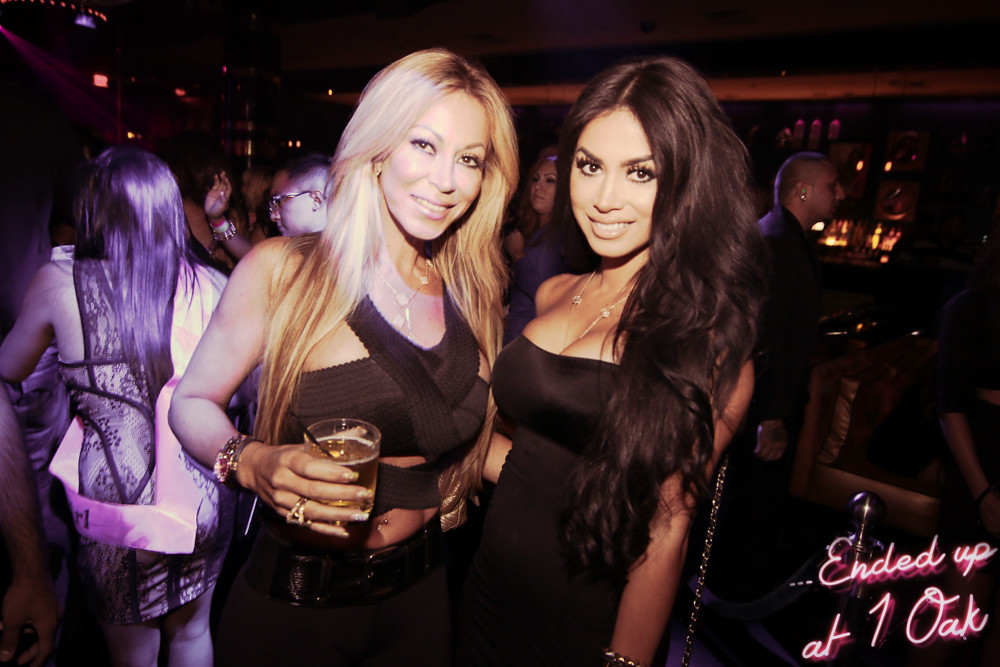The photograph depicts two women at a nightclub, posing and smiling directly at the camera. The woman on the right has long brown hair flowing down to her waist and is dressed in a strapless, low-cut black dress, accessorized with a chain likely attached to a purse off-frame. She has brown eyes and carries a light skin complexion. To her left stands a woman with almost as long blonde hair, wearing a black crisscrossed shirt and black pants with a matching belt. She holds a cup with a thin black straw, suggesting it contains an alcoholic drink. Both women, appearing to enjoy the ambiance, are at the center of the image. The background teems with other patrons, indicating a lively club scene. The overall setting seems dim but is well-illuminated by the camera’s flash, vividly capturing the image in color. At the bottom right corner of the photo, a neon sign-style text reads, "Ended up at One Oak."